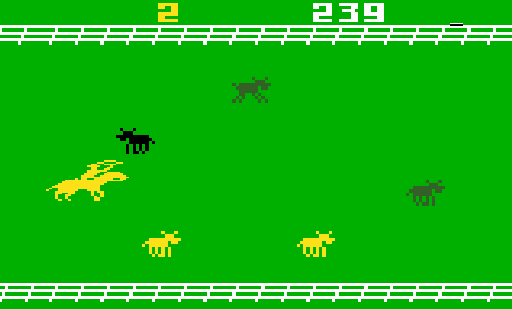This image appears to be a screenshot from an old video game, likely from early systems like the original Nintendo or Atari 2600, characterized by its simplistic, pixelated graphics. The background is a bright, light green, stretching across the entire scene. At the very top, near the center, the numeral '2' is displayed in yellow on the left side, while '239' is in white on the right. 

Prominently, two long, white fences run horizontally across the frame—one positioned at the top and another at the bottom, creating a boundary-like visual. In the center of the image is a primitive rendition of a yellow cowboy riding a yellow horse and holding a lasso, indicative of the game's objective, possibly to lasso cattle. 

Surrounding the cowboy are small, pixelated silhouettes of various animals: two are gray, two are yellow, and one is black, each appearing to resemble cows or possibly deer. The image encapsulates the nostalgic aesthetic of early video games, with its minimalistic design and limited color palette.